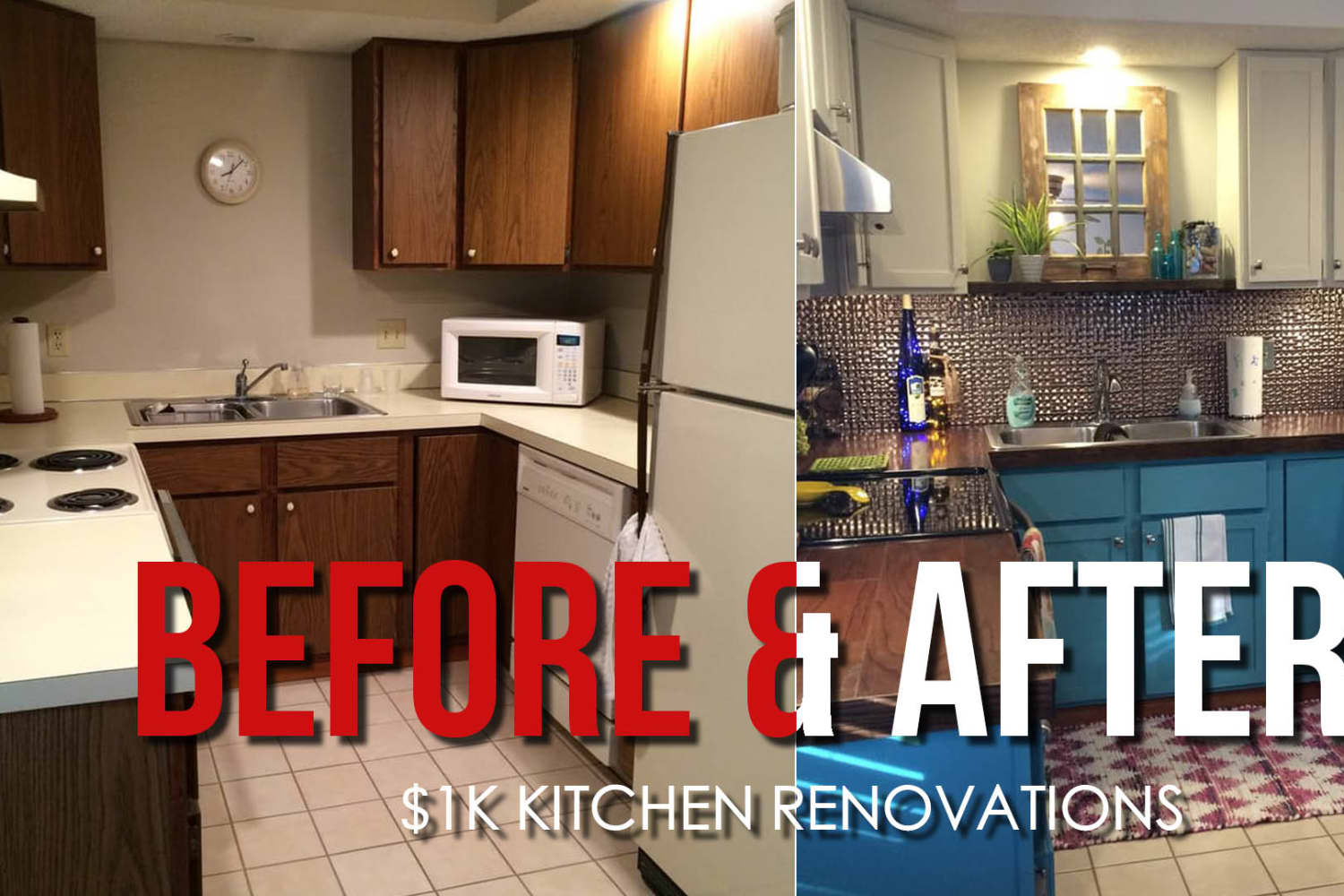The image showcases a side-by-side comparison of a kitchen before and after a renovation, prominently labeled with "Before" in red and "After" in white. Below this main text, it states "$1,000 Kitchen Renovations" in bold white font with a black outline. On the left side, the "Before" image depicts a kitchen reminiscent of the early 90s or 80s, featuring dark brown wooden cabinetry, white appliances, and an overall minimalistic design with light cream-colored and white countertops that appear somewhat outdated. The "After" image on the right reveals the same kitchen transformed with a more vibrant and modern aesthetic. It boasts glitzy, boho-chic elements, including a metallic backsplash behind the sink, better lighting, and a new stove. The countertops are now darker, adding a touch of sophistication, and there's a mirror-like window set over the sink with an accompanying light and shelf, enhancing the room's brightness and space. The overall look is a striking contrast to the original, with a more glamorous and contemporary appeal.